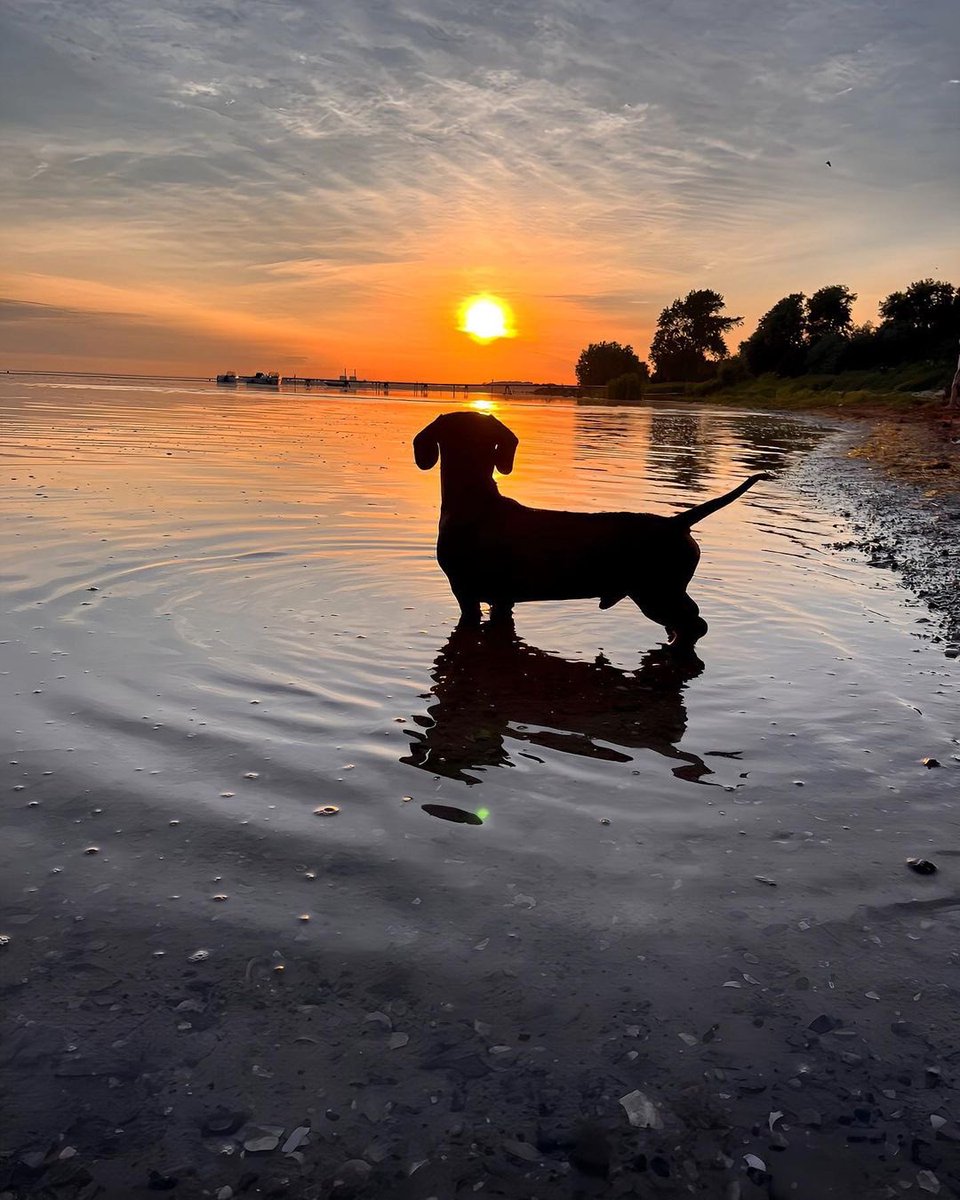The image features a silhouette of a short-legged, likely miniature dachshund standing in very shallow water, scarcely reaching the midpoint of its legs. The dog's tail is pointed upwards as it looks off to the side, casting a reflective shadow in the somewhat grimy water, which also contains submerged leaves and some visible ripples around the dog’s legs. The scene is set at dusk, with a gradient sky transitioning from dark blue above to orange near the horizon, caused by the setting sun. Shadows from the sun are visible behind several clouds. To the right of the shore, there is a row of trees and a distant pier extending into the water. The background captures a tranquil yet slightly murky lake or pond environment with the sun casting long shadows across the scene.